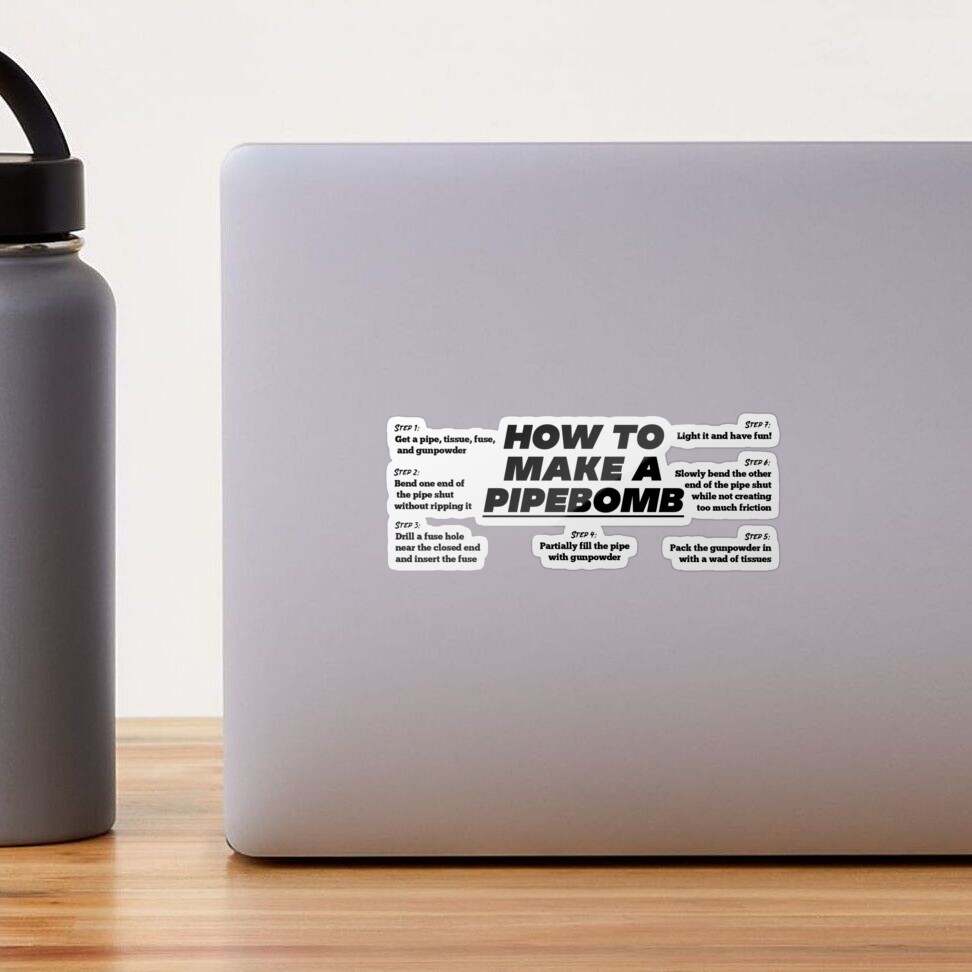The image captures a light-colored, blonde wood desk, reminiscent of a school desk, set against a white wall. On the left side of the desk, there is a vertically-cut view of a dark gray metal water bottle with a black screw-on lid. Positioned to the right of the water bottle is a lighter gray laptop, possibly an Apple product, with a conspicuous sticker that reads, "How to Make a Pipe Bomb." Surrounding this central text on the sticker, there are detailed step-by-step instructions outlining the process, enumerated from 1 to 7, although the specifics of these steps are obscured or unreadable.